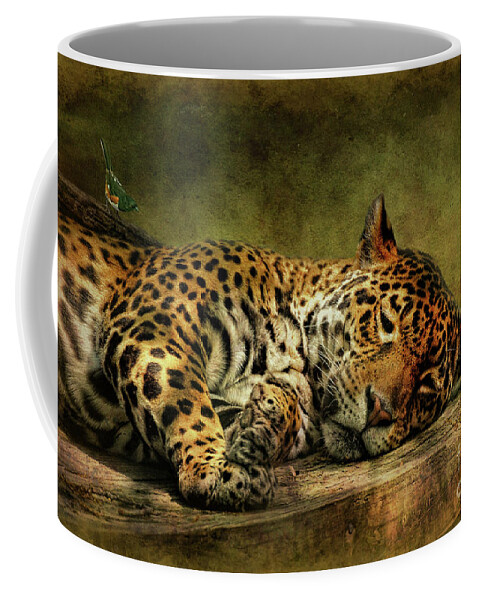A photograph of a standard cylindrical mug with a white handle, partially visible on the left side, and a white interior. The entire outer surface of the mug features a detailed, full-cover design of a resting leopard with orange fur, black spots, and beige highlights around its nose, chin, and belly. The leopard, shown from the head to the front paws and part of the stomach, appears to be lying on a piece of wood. Next to it, a small greenish-yellow bird stands, looking towards the leopard. The backdrop of the design is made up of a textured mix of green, orange, and brown, transitioning to darker shades towards the top, giving the mug a three-dimensional, almost painting-like appearance. The background outside of the mug is white, making the mug's artwork stand out prominently.